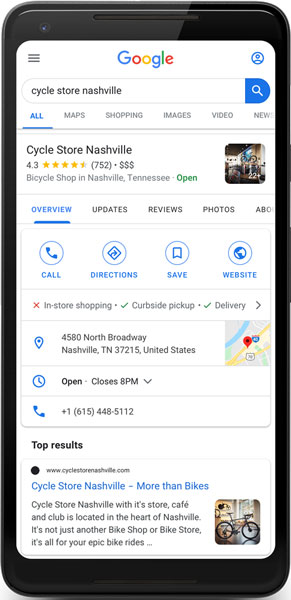A sleek, black cell phone is pictured, showcasing both its physical design and its active screen. The device features an ultra-thin speaker positioned at the top center. The screen displays a Google Search page with a clean, white background. Centered at the top is the recognizable "Google" title, just above the search bar that contains the text "Cycle Store Nashville". The search results indicate the store has a rating of 4.3 stars based on 752 reviews, and it is marked with three dollar signs, suggesting it is on the pricier side. The listing confirms it is a bicycle shop located in Nashville, Tennessee, and appears to be open at the time the screenshot was captured. Below these details, four buttons are visible: Call, Directions, Save, and Website. Further down, the address and phone number of the store are also displayed.